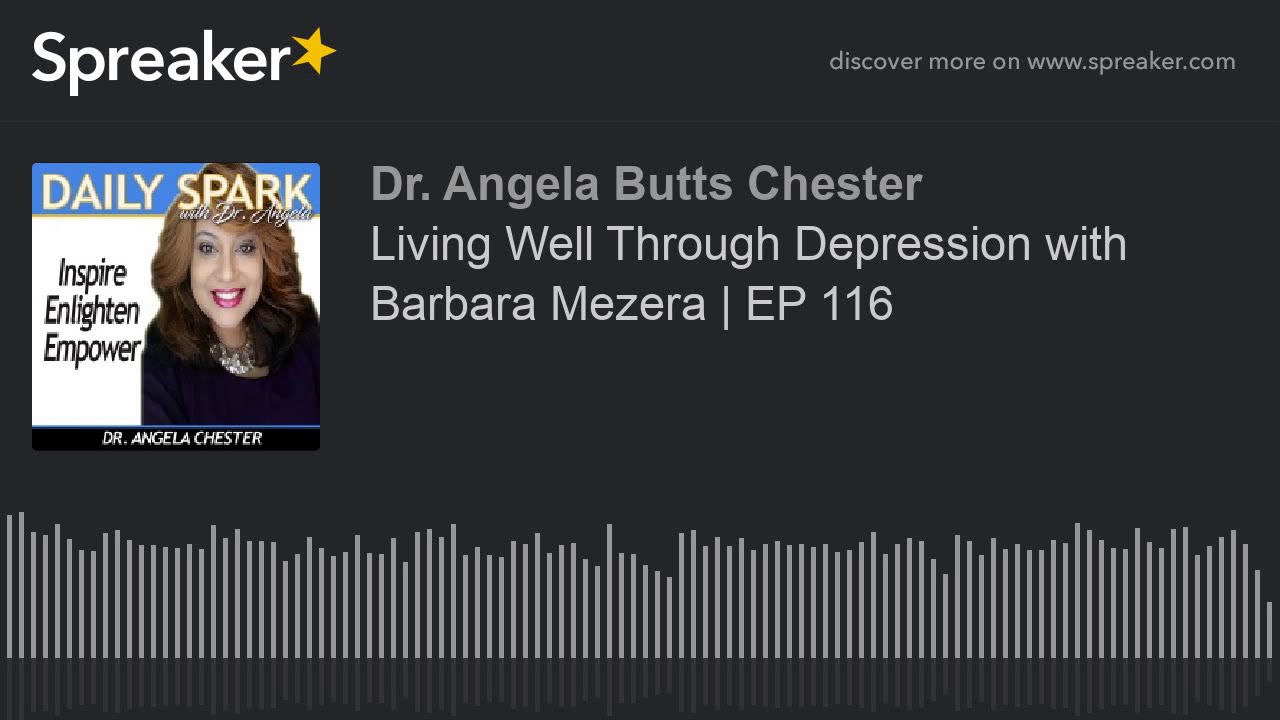The image appears to be a digital advertisement, possibly a screenshot from a music or podcast app, featuring the promotional material for an episode. The background is a dark gray color, almost black. In the upper left corner, the text "Spreaker" is displayed in white letters with a yellow star next to it. On the upper right corner, it says "discover more on www.spreaker.com" in small white letters.

On the left side of the image, there is a square with a blue highlighted section that reads "Daily Spark." Inside this square is an image of a light-skinned woman with wavy, blonde-brown hair draped over her shoulders. She is wearing a dark blue top and a large, silver necklace. Her lips are distinctly pink, and she appears to be smiling at the camera. Next to her image, there are motivational words in white text: "Inspire, Enlighten, Empower," and at the bottom, it reads "Dr. Angela Chester."

At the center of the image, larger white text states "Dr. Angela Butts Chester." Below this, in thinner white letters, it reads "living well through depression with Barbara Mezira." Further down, it specifies "Episode 116" in uppercase letters. At the very bottom of the image, there are vertical white lines that resemble sound waves or volume indicators, suggesting audio content.